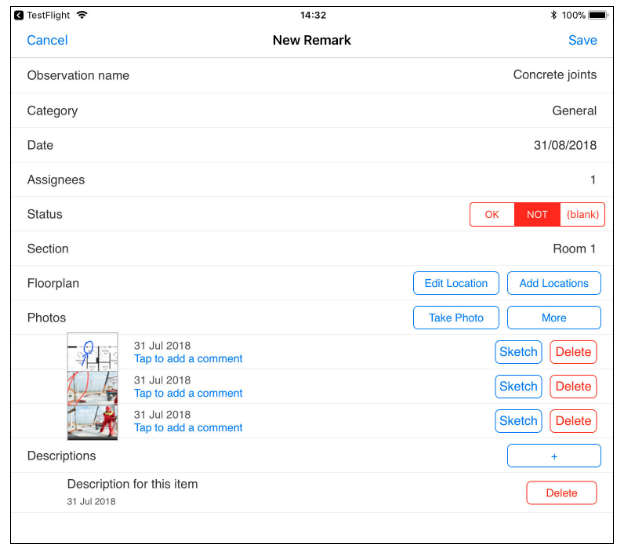This image features a white background with various text elements and icons. 

In the top left corner, the words "Test Flight" are displayed alongside a wireless connection icon. Centrally at the top, the number "1432" is prominently shown. The top right corner contains several icons: Bluetooth, a full battery indicator, and "100%."

Below these icons, the word "Cancel" appears in blue. Predominantly in the center of the page, "New Remark" is written. On the right side in alignment with this, the phrase "Concrete Joints" is visible, while on the left side, "Observation Name" is noted.

Aligned to the left are several categories listed vertically:
1. "Observation Name"
2. "Category" – with "General" directly across from it on the right
3. "Date" – paired with "31.08.2018" on the right
4. "Assignees" – with "1" noted on the right
5. "Status" – marked as "Not"
6. "Section" – linked with "Room One" on the right 
7. "Floor Plan" 

Below the categories, the term "Photos" is written.

Beneath these texts, a blurry hand-drawn stick figure is displayed atop some indistinct text, labeled with the date "31 July 2018." A prompt "Tap to add a comment" is noted underneath this.

Below this hand-drawn element, there is a photograph that is very blurry, making it difficult to identify its outdoor subject matter. The date "31 July 2018" is also present beside this image.

The image concludes with another photograph showcasing a person dressed in red on the right side, also annotated with the date "31 July 2018."